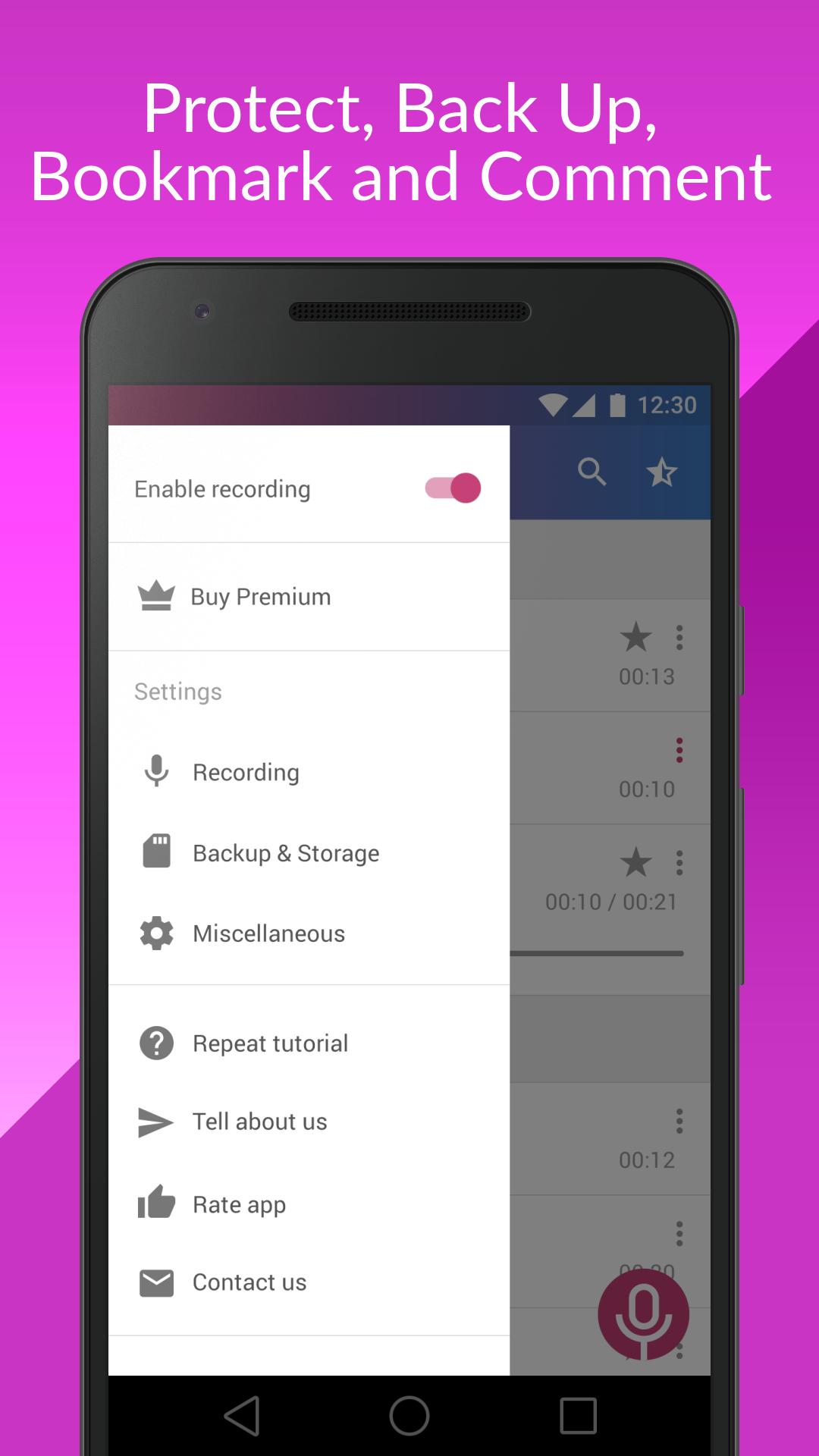The ad features a rectangular graphic, roughly the size of a phone screen, with a split background consisting of two shades of purple—lighter purple at the top and darker purple at the bottom. In the top portion, bold white text prominently displays the words: "Protect, Back Up, Bookmark, and Comment."

Centrally positioned within the purple background is an image of an Android phone, identifiable by its distinctive navigation buttons at the bottom. The phone's screen shows an overlay and underlying application interface. The overlay is a white pop-up message that reads "Enable recording," accompanied by a toggle switch set to 'off.' Directly below this, there's an option that says "Buy Premium."

Underneath the pop-up, the screen displays various setting options, each paired with a relevant icon. The settings include:

- **Recording**: Illustrated with a microphone icon.
- **Backup and Storage**: Not described in detail.
- **Miscellaneous**: Not described in detail.
- **Repeat Tutorial**: Marked with a gray box featuring a question mark.
- **Tell About Us**: Not described in detail.
- **Rate App**: Indicated with a thumbs-up icon.
- **Contact Us**: Represented by an envelope icon.

This highly detailed ad layout showcases the features and premium options of a mobile app, emphasizing functionality such as recording, data backup, and user engagement.